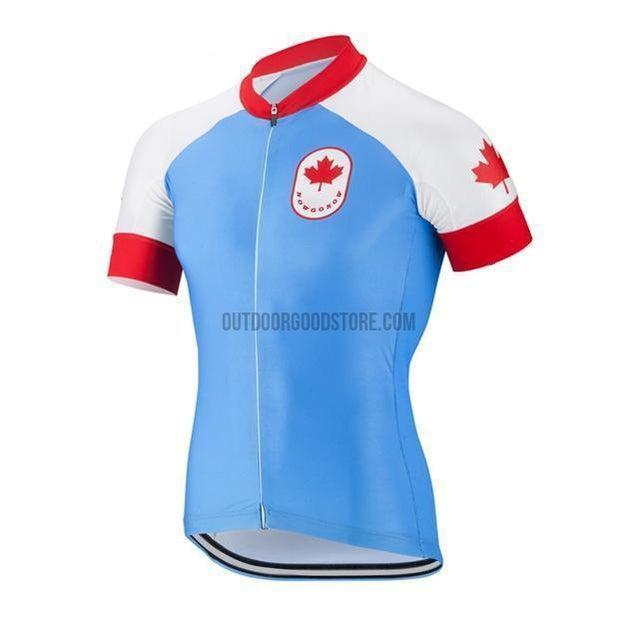This detailed image showcases a Canadian athletic or cycling uniform shirt prominently featuring the iconic red maple leaf. The shirt is primarily light blue, with short raglan-style sleeves that are white, accented by red cuffs at the ends. The collar also features a red band that matches the sleeve trims, creating a cohesive design. A standout feature is an illustration of a red maple leaf emblazoned on the left shoulder. The shirt zips up the front, leading to an oval-shaped emblem on the left chest, which contains a red maple leaf against a white background and some unreadable text underneath. The backdrop of the photo is white, subtly marked with the word "OutdoorGoodstore.com".